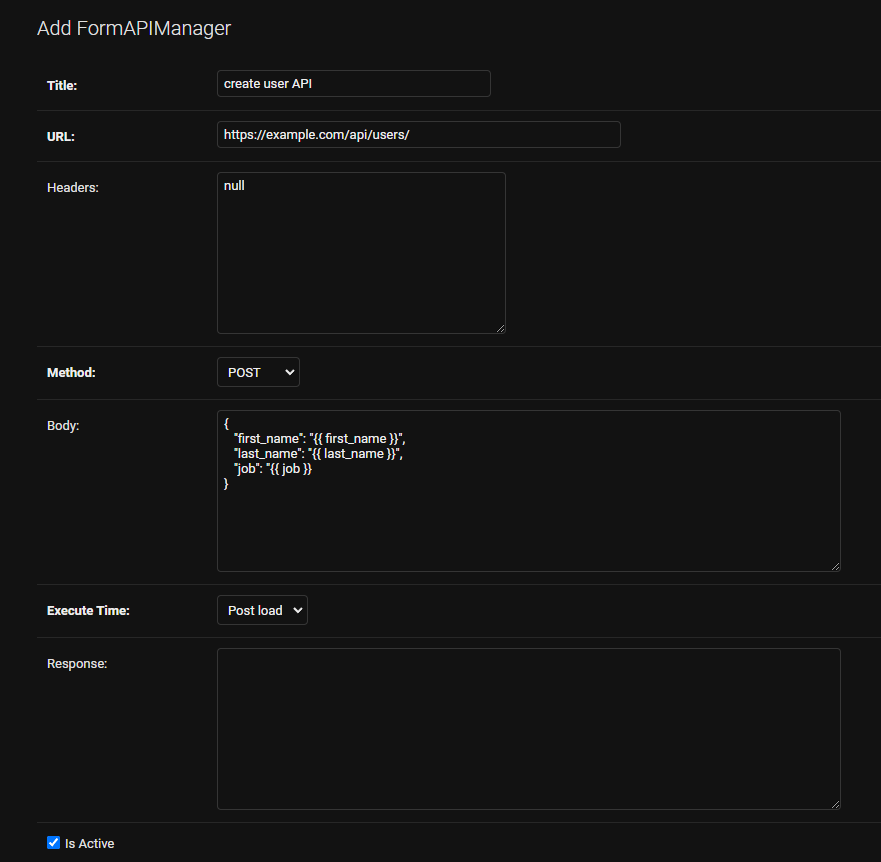This vertical rectangular image features a dark black background. Situated in the upper left-hand corner, the text "Add Form API Manager" is displayed prominently in white font. 

Directly below, a series of labeled sections are written in bold white font, each with an associated input field or dropdown menu accompanied by faint horizontal lines for separation. These sections and fields are described as follows:

1. **Title:** 
   - **Label:** "Title:"
   - **Field**: Positioned about a third of the way from the left, the field contains the text "Create User API."

2. **URL:**
   - **Label:** "URL:"
   - **Field:** Contains the web address "https://example.com/api/users/."

3. **Headers:**
   - **Label:** "Headers:"
   - **Field:** A large horizontal rectangular box displaying the word "NULL."

4. **Method:**
   - **Label:** "Method:"
   - **Field:** A smaller rectangular box with a dropdown menu displaying the word "POST" in all caps.

5. **Body:**
   - **Label:** "Body:"
   - **Field:** Contains what appears to be computer language or code.

6. **Execute Time:**
   - **Label:** "Execute Time:"
   - **Field:** A small box with a dropdown menu displaying the option "Post Load."

7. **Response:**
   - **Label:** "Response:"
   - **Field:** An empty, large horizontal rectangular box.

At the very bottom of the image, a square turquoise button featuring a white checkmark and the text "is active" is situated, indicating some form of toggle or activation option.

The entire layout is cleanly separated by thin horizontal lines, organizing the sections and providing clarity and order for each element on the page.